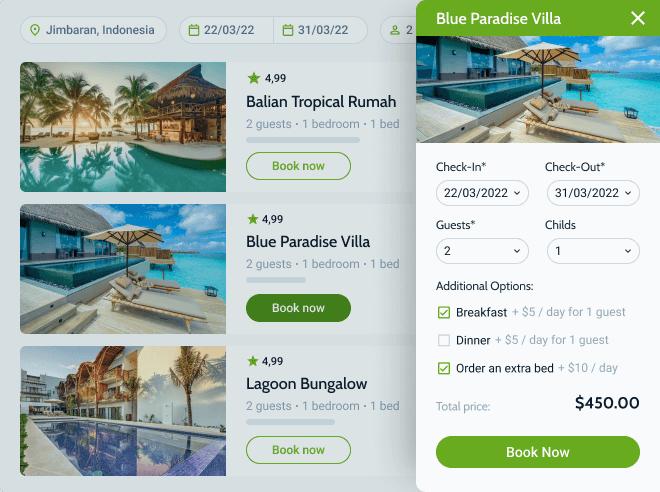A user is browsing a booking website, looking at options for a hotel stay in Jimbaran, Indonesia for the dates 22nd March 2022 to 31st March 2022. The available accommodation choices include Balian Tropical, Rama Blue Paradise Villa, and Lagoon Bungalow. They have selected the "Blue Paradise Villa", as indicated by a highlighted section on the web page. 

The "Blue Paradise Villa" option features a background with a lime-green color and blue text. At the top of the selection window, there's an image showcasing an elaborate outdoor pool adjacent to a beach—a combination that might seem redundant but offers a luxurious appeal. The booking details specify check-in on 22nd March 2022 and check-out on 31st March 2022, with a total of two adults and one child as guests. 

Additional options provided include breakfast at $5 per day for one guest, which is selected, but dinner at the same price per guest and an extra bed at $10 per day are not chosen. The total cost for the stay amounts to $450, which is noted as quite expensive for Indonesia. The detailed selection showcases the high-end nature and cost of the stay, emphasizing the premium experience the user is opting for.